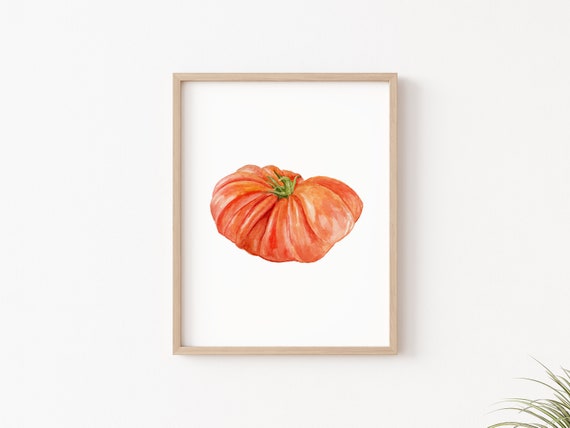This photograph displays a framed picture hanging on an off-white wall tinged with a hint of purple. The picture, contained within a plain wooden frame that is light brown with a nearly pinkish hue, features a white background. In the center of the image is what appears to be a shriveled or dried tomato—or possibly a pumpkin—characterized by its wrinkled, folded texture, and a green stem at its middle. The tomato/pumpkin displays a mix of hues, with rose peach tones and occasional red accents in its creases, giving it a waxy sheen. In the lower right corner of the photograph, the edges of a plant with long, slender leaves are visible, suggesting an indoor setting for this art piece. The overall image is slightly wider than it is tall, emphasizing the expansive feel of the scene.